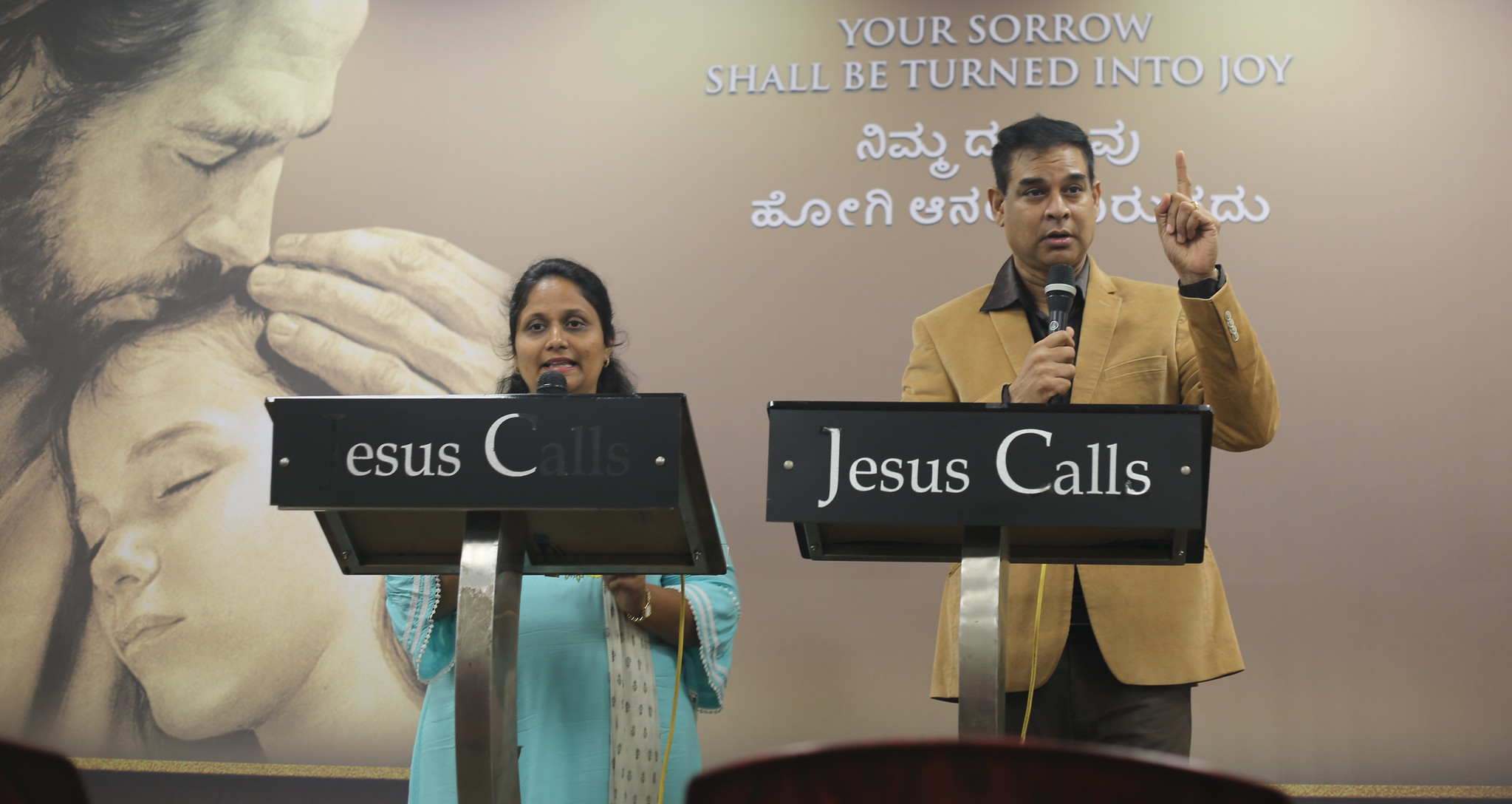In this detailed image, two Indian speakers are positioned at the front, each standing behind a silver and black podium inscribed with the words "Jesus Calls." The scene appears to be set in a church or exhibition hall, with a background projection of a serene Jesus tenderly holding and kissing a little girl’s head, accompanied by the comforting words, "Your sorrow shall be turned into joy." 

The man on the right, dressed in a gray suit jacket over a black shirt and dark pants, is animatedly pointing upwards with his left hand while holding a microphone in his right, indicating that he is speaking. To his left, the woman stands at a lower podium due to her shorter stature. She is adorned in a traditional Indian dress of a light blue-teal color with off-white trimming, and has long black hair. She too holds a microphone, fully engaged in delivering her message as suggested by her expressive face. The harmonious color coordination and the inclusive religious theme create a visually impactful and spiritually resonant scene.